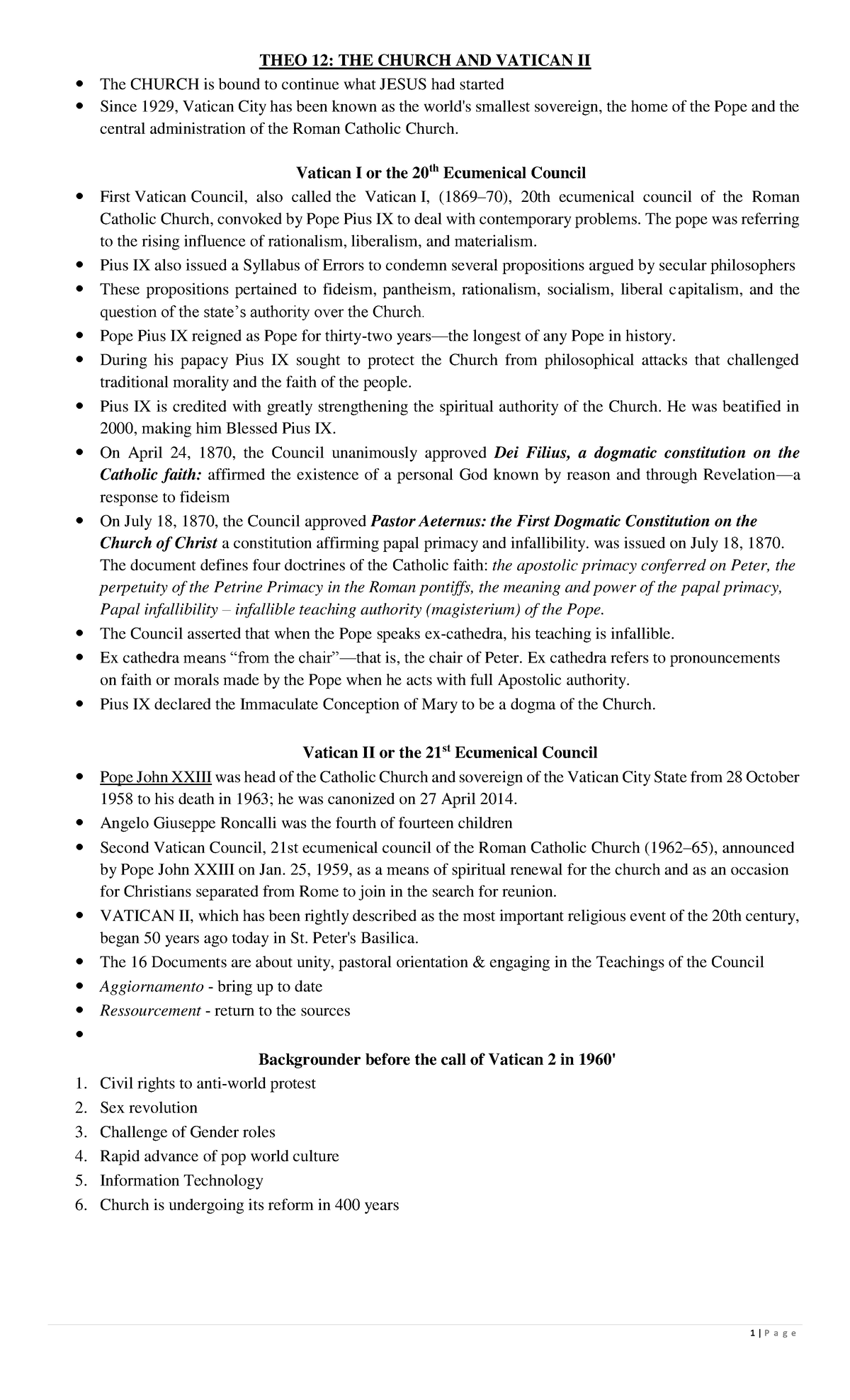This image captures a segment from a newsletter or an email discussing church-related topics, specifically focusing on the Vatican and its councils. The background is white, adorned with substantial amounts of black text. The content is heavily centered on religious discourse and is organized with bullet points to cover various topics.

The layout includes small circular black dots on the left side marking each bullet point. These points consist of concise sentences or short paragraphs, each separated by a bit of whitespace, ensuring clarity and readability. 

Structured titles guide the reader through the content:
1. "The O-12, the Church and the Vatican" - potentially indicating a Roman numeral II.
   - "Vatican I or the 20th ECUMENICAL Council"
   - "Vatican II or the 21st ECUMENICAL Council"

The section concludes with:
- "Backgrounder Before the Call of Vatican II in 1960" which segues into a list of six numbered points, providing additional context or closing remarks related to the Vatican II council preparation phase in 1960. 

Each of these elements collectively offers a detailed and structured overview of the subject matter, making it accessible for readers engaging with the religious and historical content provided.